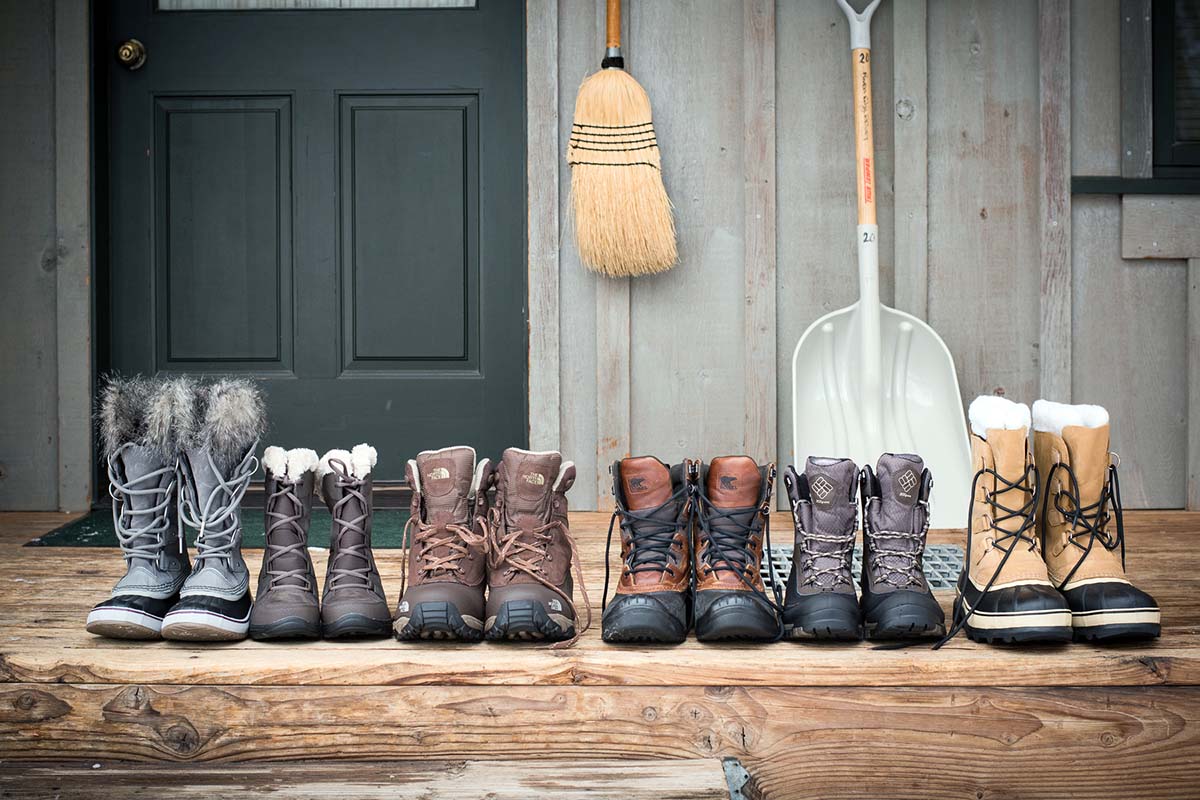In this daytime outdoor photograph, we see a wooden porch with six pairs of boots carefully aligned. The porch is part of a house with gray walls and a dark green door at the center, accented by a gold handle. A green mat lies in front of the door. Hanging on the wall beside the door is a broom, and a snow shovel with a gray scoop and wooden handle rests against the house. The boots, presumably for snow and hiking, showcase a variety of styles and colors. From left to right, the first pair is gray with fur trim and gray laces. Next, there's a smaller pair of dark brown boots with brown laces and white lining. Following that is a pair of light brown boots with black tips. The subsequent pair features reddish-brown boots with black tips and laces. Further along, there's a pair that appears purplish-brown with black bottoms. Finally, on the far right are tall, light brown boots with fleece lining at the top and black laces running down to black soles.